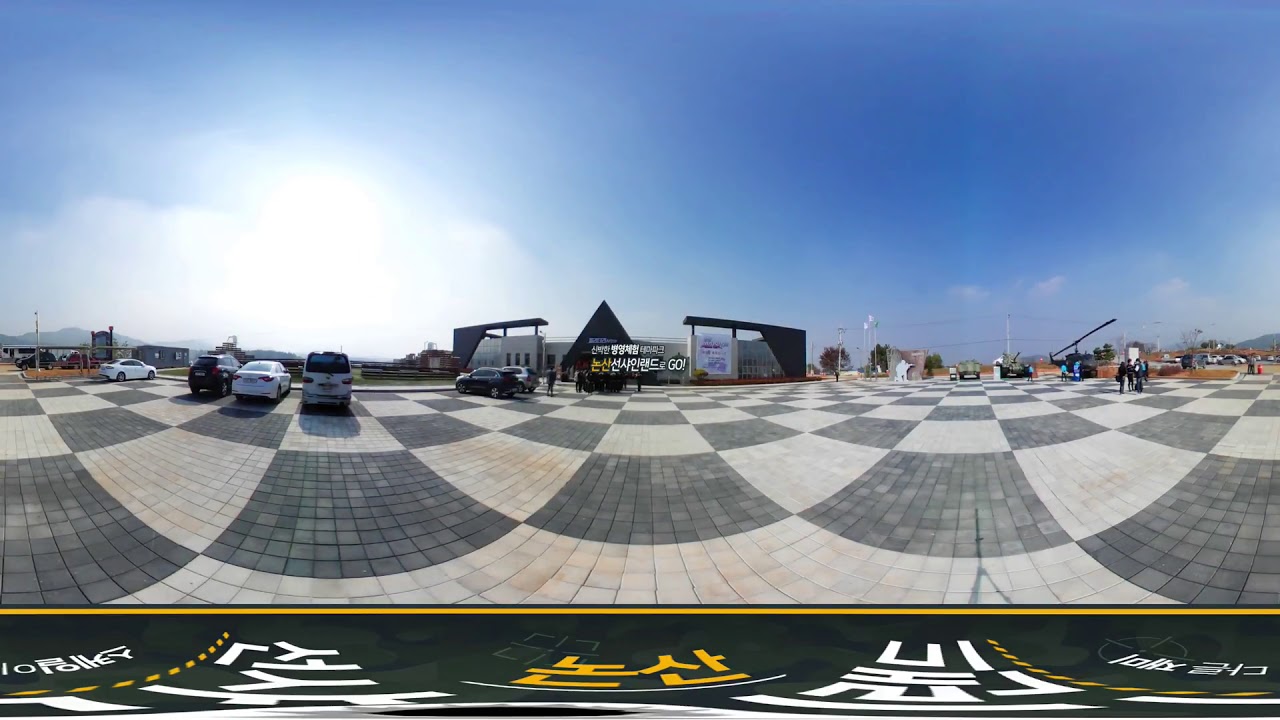The image depicts a panoramic view of a shopping center's parking area with a distinctive gray and beige checkered pavement pattern. Cars are predominantly parked on the left-hand side of the image. The center of the image features a white and gray building with a triangle-shaped entranceway. The road is characterized by a unique pattern that, while appearing checkered, consists of arcs and square-like shapes. At the bottom of the image, there is a line of yellow and white text in a foreign language, possibly Japanese or another Asian script, which is not fully legible. In the background, electrical lines, streetlights, and small trees dot the horizon. The sky takes up almost half of the image, showcasing a very blue expanse with a few clouds and a bright white area on the left side, possibly with the sun shining. There are faint, indistinct shapes of people and vehicles, including what looks like a ghostly figure of a shooter, perhaps computer-generated, hinting at a gaming overlay.